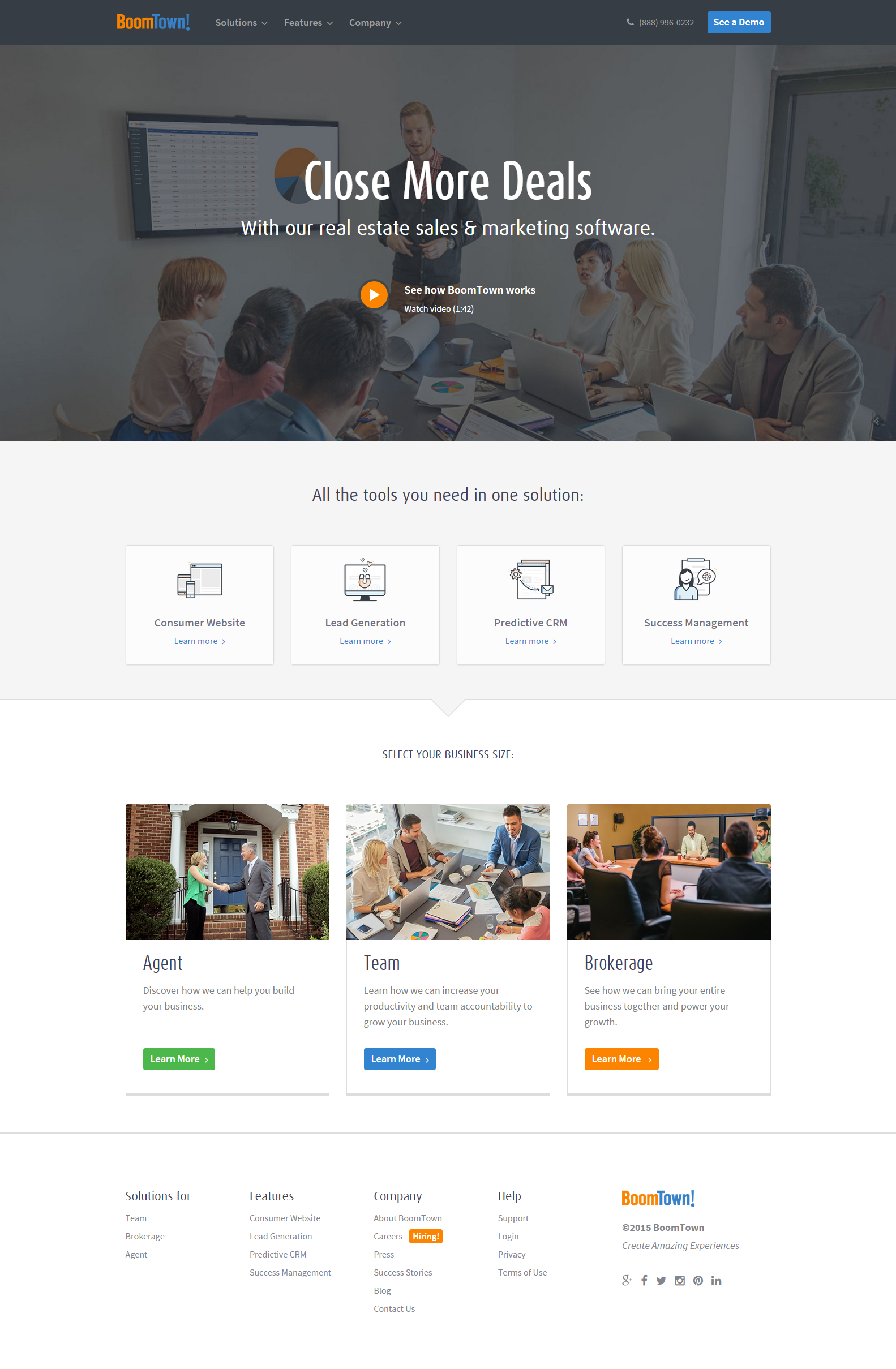A screenshot of a website dedicated to real estate sales and marketing software prominently displays the headline "Close More Deals" at the top center. Directly below, the tagline reads, "With Our Real Estate Sales and Marketing Software." Beneath this, a subheader promises, "All the Tools You Need in One Solution." The main section showcases four distinct examples of these integrated tools. Farther down, the page is segmented into three categories: Agent, Team, and Brokerage, each seemingly designed to cater to different user needs within the real estate industry. The bottom section of the webpage contains the usual footer elements, completing the informative and comprehensive layout of the site.